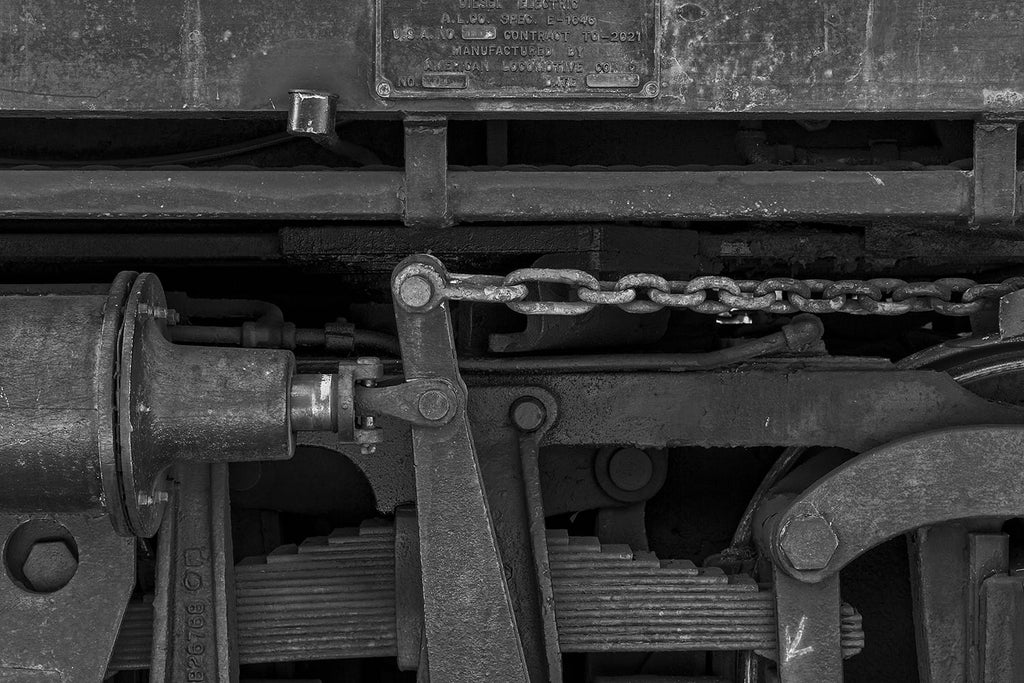This detailed black-and-white photograph captures a close-up view of an intricate mechanical contraption, most likely part of a train or locomotive. The image showcases an array of interlocking mechanisms, including numerous levers, bolts, gears, and chains, all crafted from dark gray metal and iron. Central to the shot is a robust metal chain that extends from the middle of the photograph towards the right side, possibly connected to or drawing power from a piston system. A prominent plaque, situated at the top of the assembly, bears raised lettering that partially reads, "USA contract TO 2021 manufactured by American Locomotive," though some of the text is worn and hard to decipher. Additionally, a piece of metal featuring a white arrow pointing down and to the left is visible in the bottom right corner, emphasizing the detailed and functional nature of this historical machine.